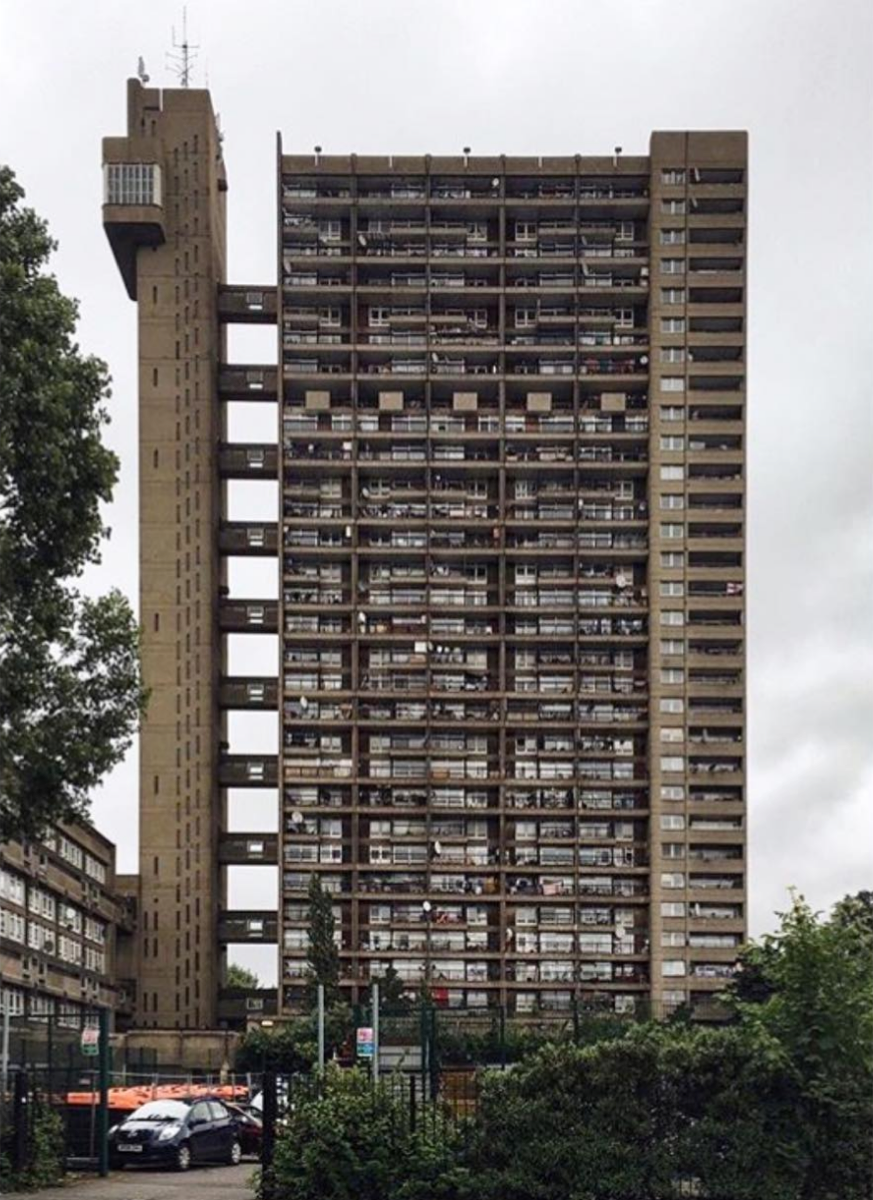The image depicts a tall, somewhat unremarkable apartment building standing approximately 20 to 30 stories high, set against a cloudy gray sky in an urban environment. The building comprises two distinct parts: a main residential structure to the right and a thinner vertical tower to the left, with connecting breezeways linking the two every few stories. The building features outdoor balconies or patios, some of which have visible furniture and people. In the foreground, there's a parking lot enclosed by a fence, containing a blue car and several other dark-colored cars. The scenery includes shrubs, greenery, and part of a tree on the left side. An open gate and some foliage further accentuate the setting, and another building, possibly a factory, is partially visible in the lower left background. The left tower of the building also has an antenna on top, adding to the overall structural detail.